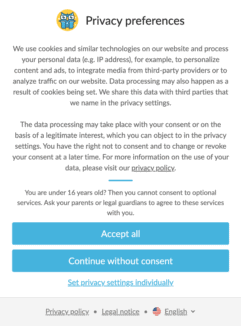The image presents a detailed overview of privacy preferences for a website. It informs users that cookies and similar technologies are used to process personal data, including IP addresses, to personalize content and advertisements, integrate third-party media, and analyze website traffic. The image highlights that data processing may result from cookies being set, and that this data is shared with third parties named in the privacy settings. It also mentions that data processing may occur either with the user's consent or based on legitimate interest, which users can object to in the privacy settings. The rights of users are emphasized: they may choose not to consent, and they can change or revoke their consent at any time. Additionally, users under 16 years old are instructed to seek consent from their parents or legal guardians for optional services. Options to either "Accept," "Continue without Consent," or "Set Privacy Settings Individually" are provided, guiding users in managing their privacy choices. For further details on data usage, users are directed to the privacy policy.